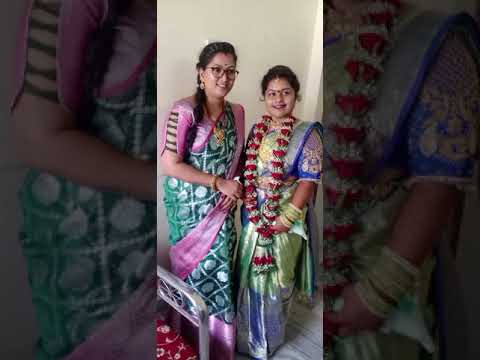The image is a vertical cell phone picture featuring two Indian women posing against a bright white wall with grey carpet beneath. Behind them, the same image is magnified and faded, focusing on their torsos and hips. The woman on the left is taller, with braided black hair draped over her shoulder and wearing glasses. She is adorned in a traditional Indian dress with a green pattern and a purple sash. The woman on the right is shorter, with her black hair pulled back, and she wears a bluish-green dress with a green sash. Both women have red dots in the center of their foreheads, indicating bindi, and the woman on the right accessorizes with a large, possibly floral-designed necklace. In the background, to the left, there is also the image of a metal footboard with a red blanket.